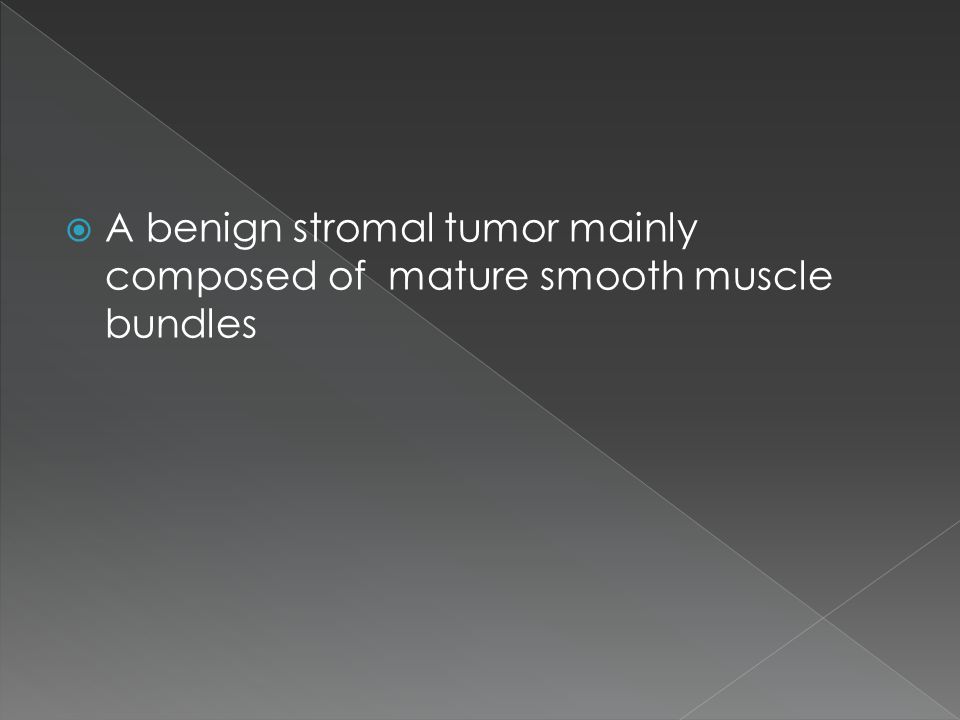The image depicts a presentation slide with a background divided into four triangles. The background features a prominent vertical line running diagonally from the top left corner to the bottom right corner, creating two major triangles. The top right triangle is a darker gray, while the bottom left triangle is a lighter gray. Additionally, there is another diagonal line in the bottom right corner, splitting one of the triangles further, ultimately dividing the entire background into four triangles. The text on the slide, displayed in white font on a blue bullet point, reads: "A benign stromal tumor mainly composed of mature smooth muscle bundles." This text is positioned to the right of a small blue dot and appears against a flat, monochromatic background, likely indicating a computer screen or PowerPoint presentation setting.